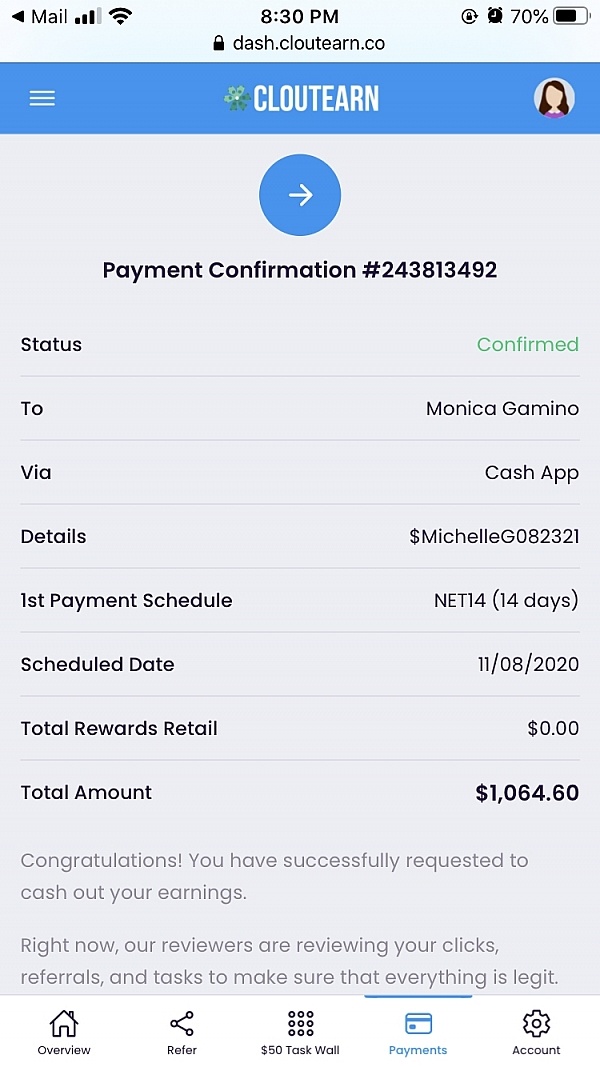The image depicts an email page from a service named "Cloutern" (spelled C-L-O-U-T-E-A-R-N), presented with white text on a blue background. A notable feature is a thumbnail of a girl with long brown hair, though this is an illustrated icon rather than a photograph. Below the thumbnail, there is a white arrow encased in a blue circle, accompanied by the label "Payment Confirmation, #243813492."

The layout includes a left-hand column with the heading "Status," which is followed by the word "Confirmed" in green on the right-hand side. The payment is directed to a Monica Gamino via Cash App. The email further provides detailed information: the amount is listed as $1064.60, with transaction details under the name Michelle G-O-82321. The email notes that the first payment is scheduled for 14 days after the listed date, which is November 8th, 2020. The "Total Rewards" section indicates a balance of zero, but the "Total Amount" confirms the sum of $1064.60.

At the bottom of the email, a congratulatory message reads, "Congratulations, you've successfully requested to cash out your earnings." This emphasizes the user's successful action in withdrawing their funds. The overall tone and detailed breakdown of information contribute to the impression of a well-documented financial transaction.